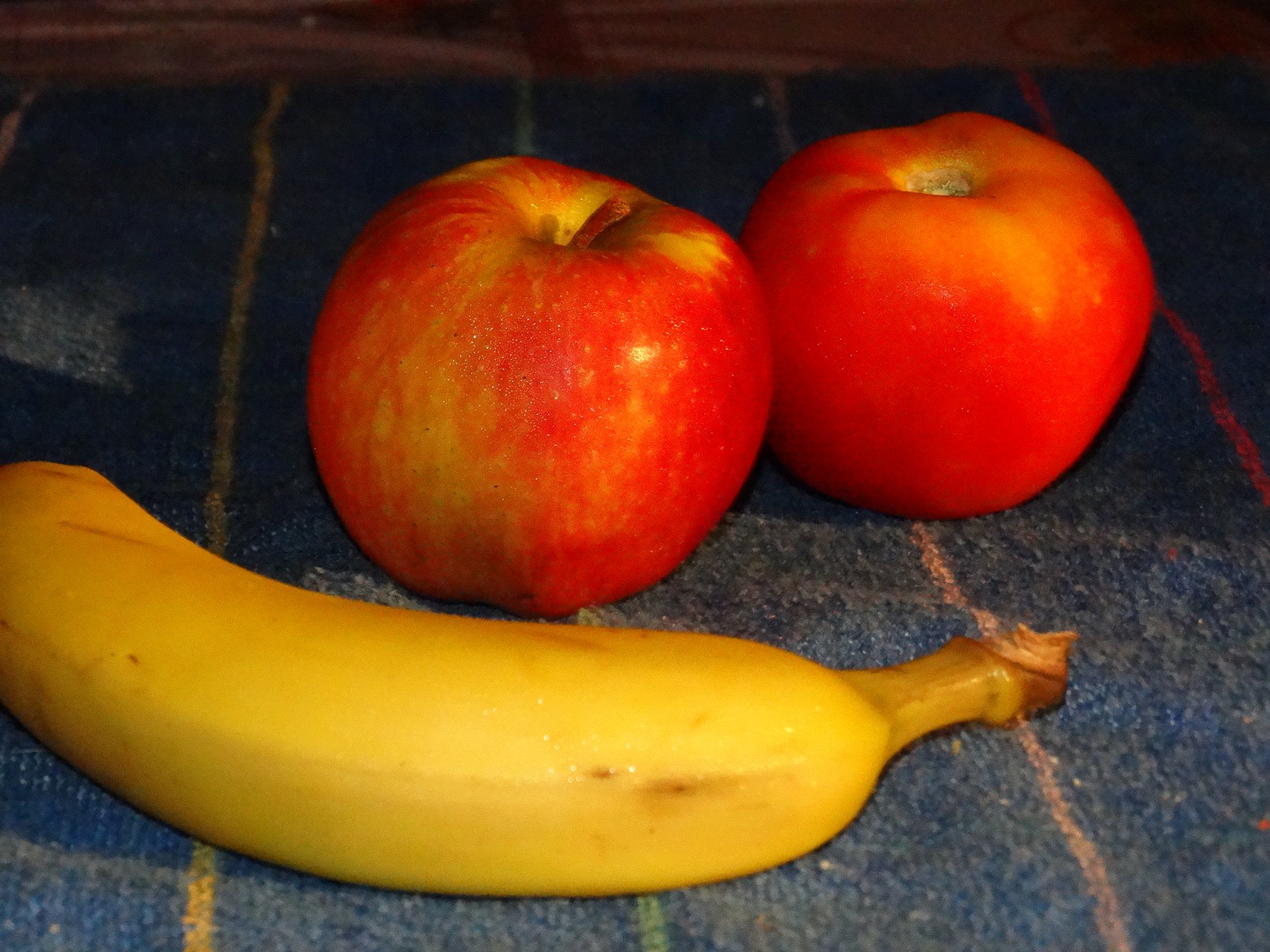A detailed indoor color close-up photograph captures three fruits arranged on what appears to be a blue cloth, possibly a placemat, atop a tabletop. In the foreground, a ripe banana lies horizontally, with its slightly brown-spotted stem pointing towards the right edge of the frame. The banana exhibits a greenish-yellow hue, leaning more towards yellow. Positioned behind the banana, to the left of center, is a ripe red apple. Its visible stem points diagonally to the right. Just behind the apple, towards the right, sits a reddish-orange tomato devoid of a stem. The upper left, right, and center background areas are predominantly dark, offering only glimpses of the blue cloth. The image is well-lit from the right side, casting subtle shadows of the fruit towards the left. Each element within the frame is sharply in focus, with no additional objects or text present in the composition.